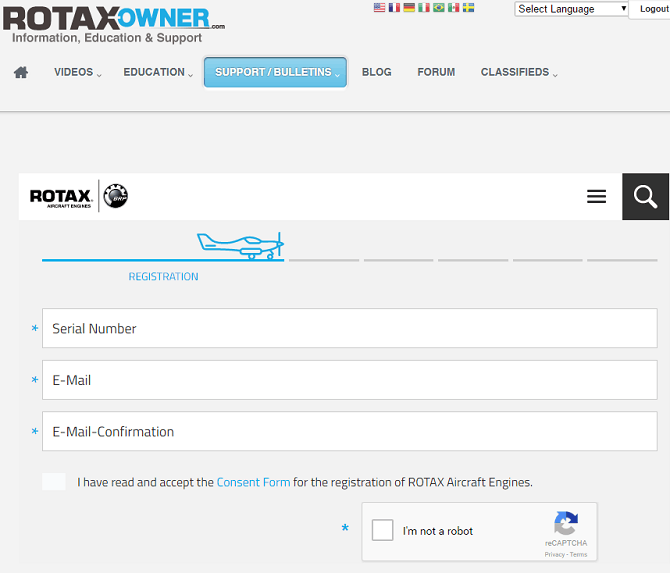Screenshot of the Rotex Owner Website Registration Page

This screenshot captures the registration page of the Rotex Owner website, presented on a predominantly white background. On the top-left corner, there's a stylized logo reading "Rotex Owner"; "Rotex" appears in gray while "Owner" is in blue, with a small ".com" beside it. Below the logo, the tagline "information, education, and support" is displayed. 

To the right, a selection of international flags allows users to choose their preferred language, and a "Logout" button is situated in the top-right corner. 

The navigation menu beneath the header consists of several options: "Home," "Videos," "Education," "Support," and "Bulletins" (the latter highlighted in blue), followed by "Blog," "Forum," and "Classified," all written in a gray font.

Centered on the page, the word "Rotex" is followed by a blue line above three horizontal input boxes labeled serial number, email, and email confirmation, each marked with a blue asterisk indicating required fields. Adjacent to these fields, there is a simple drawing of a blue airplane. 

Below the input fields, a checkbox states, "I have read and accept the consent form for registration of Rotex aircraft engines," followed by an "I'm not a robot" CAPTCHA. The CAPTCHA includes its recognizable circular rotating arrow icon in a gradient from gray to blue, with a checkbox for user interaction beside it.

Overall, the layout is minimalistic, with ample white space and a straightforward design aimed at facilitating user registration with clarity and ease.